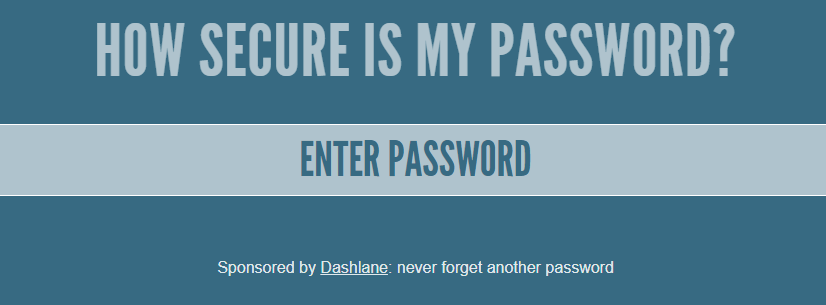The image features a password strength evaluation tool prominently displayed in the center of a dark blue background. The tool, sponsored by Dashlane, a well-known password manager, invites users to enter a password to assess its security level. The input field, situated within a gray horizontal band in the middle of the image, accommodates users as they type in various passwords. 

Upon entering a password, the tool immediately evaluates and displays its strength, ranging from "weak" for simple combinations, such as eight lowercase letters, to "strong" for more complex, robust passwords. This interactive feature is designed to educate users on the importance of creating secure passwords by incorporating diverse characters. 

Overall, the layout suggests a standalone interface, wide and user-friendly, approximately twice as wide as it is tall. Though the request to input a password may seem unusual, it serves as a practical educational tool to enhance password security awareness.